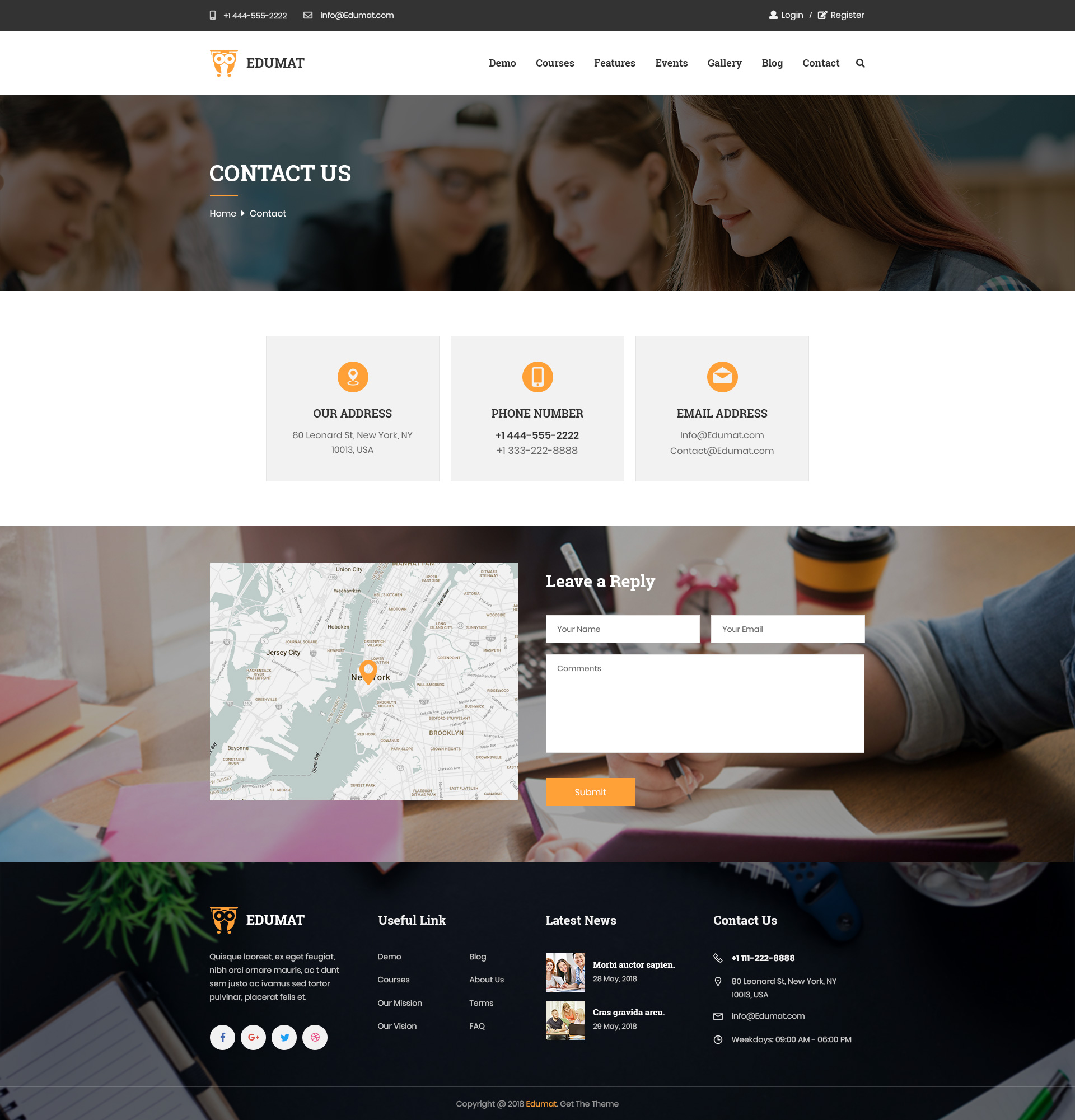The image depicts a webpage with a predominantly white and black color scheme, accented with orange icons and text. At the top, there is a black navigation bar displaying a telephone number (144-565-2222), an indistinct email address, and buttons for login and registration. Beneath this, an orange-eyed icon accompanied by the word "Edumat" can be seen, followed by navigation links for "Demo," "Courses," "Features," "Events," "Gallery," "Blog," and "Contact," alongside a search icon represented by a magnifying glass.

Below this header section, a rectangular banner features an image of students seated in the background with the text "Contact Us" and "Home." Further down, there are three information squares: the first one provides the address (80 Leonard Street, New York, NY 10013, USA), the second lists another phone number (144-555-2222), and the third displays the email address (info@edumat.com). A map showing the location is also visible in this section.

Beneath these elements, there is a "Leave a Reply" section with fields for name, email, and comments, accompanied by a submit button. At the bottom of the page, the "Edumat" name reappears, along with social media links and additional useful and contact us links.